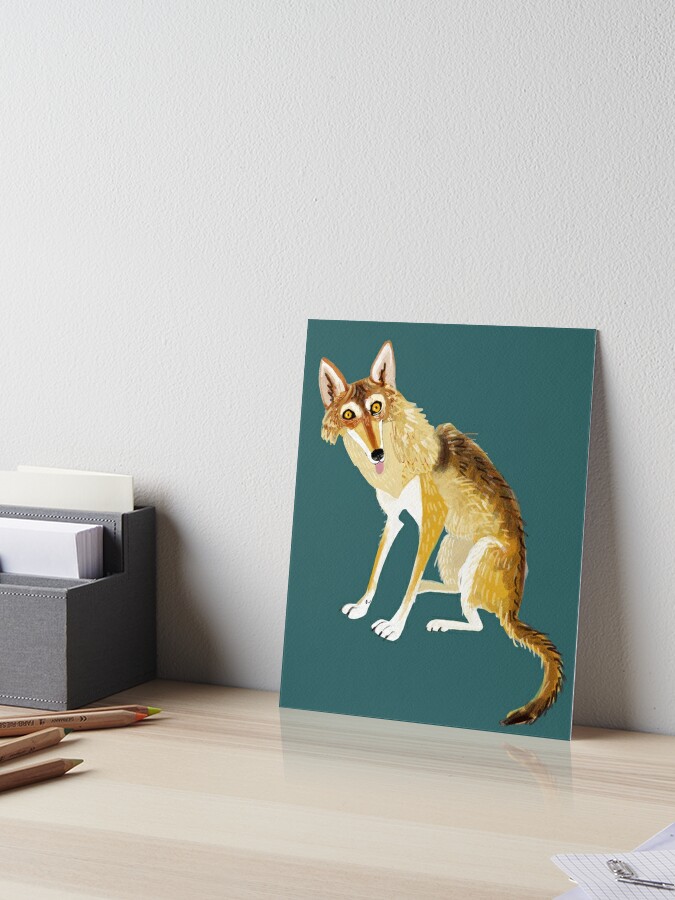The image shows a lightly-colored, wood-grain desk with a shiny lacquer finish. On the left side of the desk, there are four colored pencils in yellow, orange, blue, and white, with one of the pencils displaying some unreadable text. Beside the pencils, there is a gray, two-tiered box or organizer, housing small envelopes and casting a shadow on the white wall behind it.

To the right of the organizer, prominently displayed, is an 8 x 10 painting of a fox. The fox sits against a green background, its pink tongue sticking out, yellow eyes alert, and pointed ears perked up. The fox's breast is white, its paws are white, and its tail features dark brown with black stripes. In the bottom right-hand corner of the image, there is a piece of lined paper with a silver item resting on top, hinting at a possible artist's workspace. The desk forms a stark contrast with the off-white wall, creating a clean and organized yet creatively charged environment.